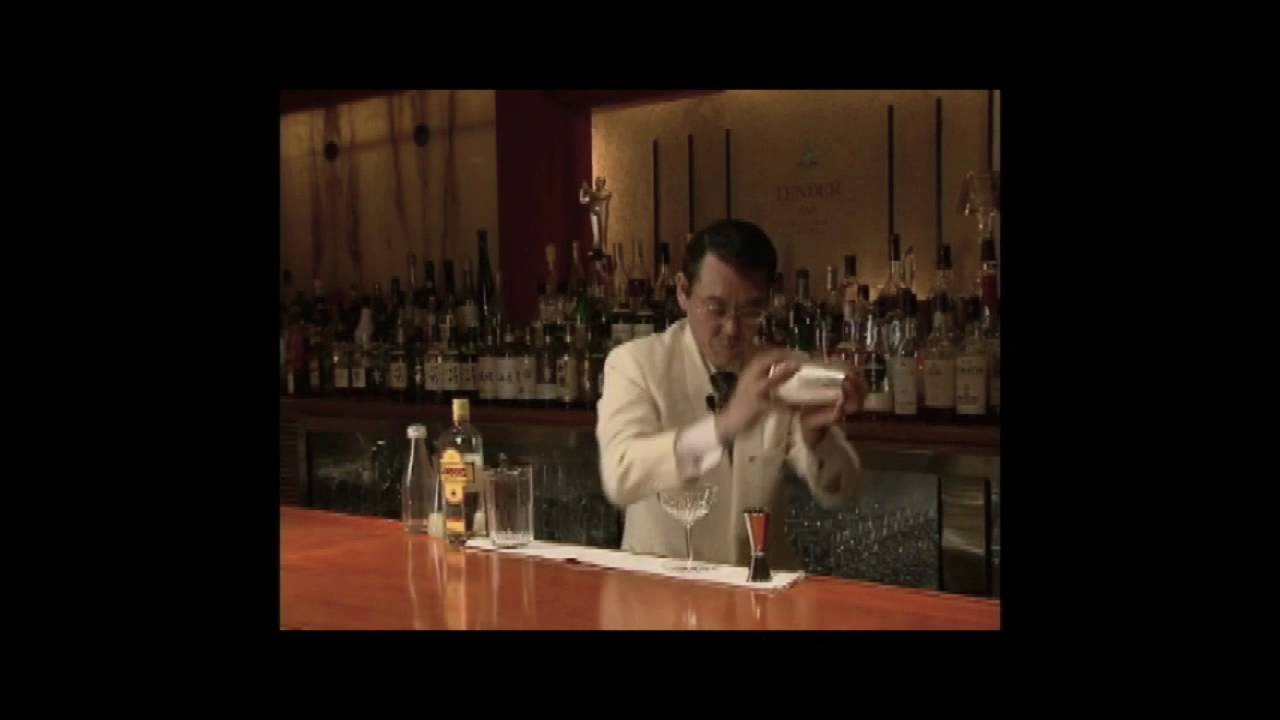In this photo, a bartender is seen skillfully shaking a silver cocktail shaker behind a wooden bar counter. He appears to be in his 50s, has short dark brown hair, and is wearing glasses. His attire includes a white tuxedo suit paired with a black tie. The setting is dimly lit with a black border framing the image, thicker on the sides than at the top and bottom. In front of the bartender, there are several items on the brown lacquered bar surface: a martini glass, a bottle of liquor with a yellow label, another glass bottle, and a regular shot glass. Behind him, rows of liquor bottles are neatly aligned on a shelf against a dark mustard-colored wall. This striking contrast between the dark background and the bartender's white attire makes for a visually compelling scene.